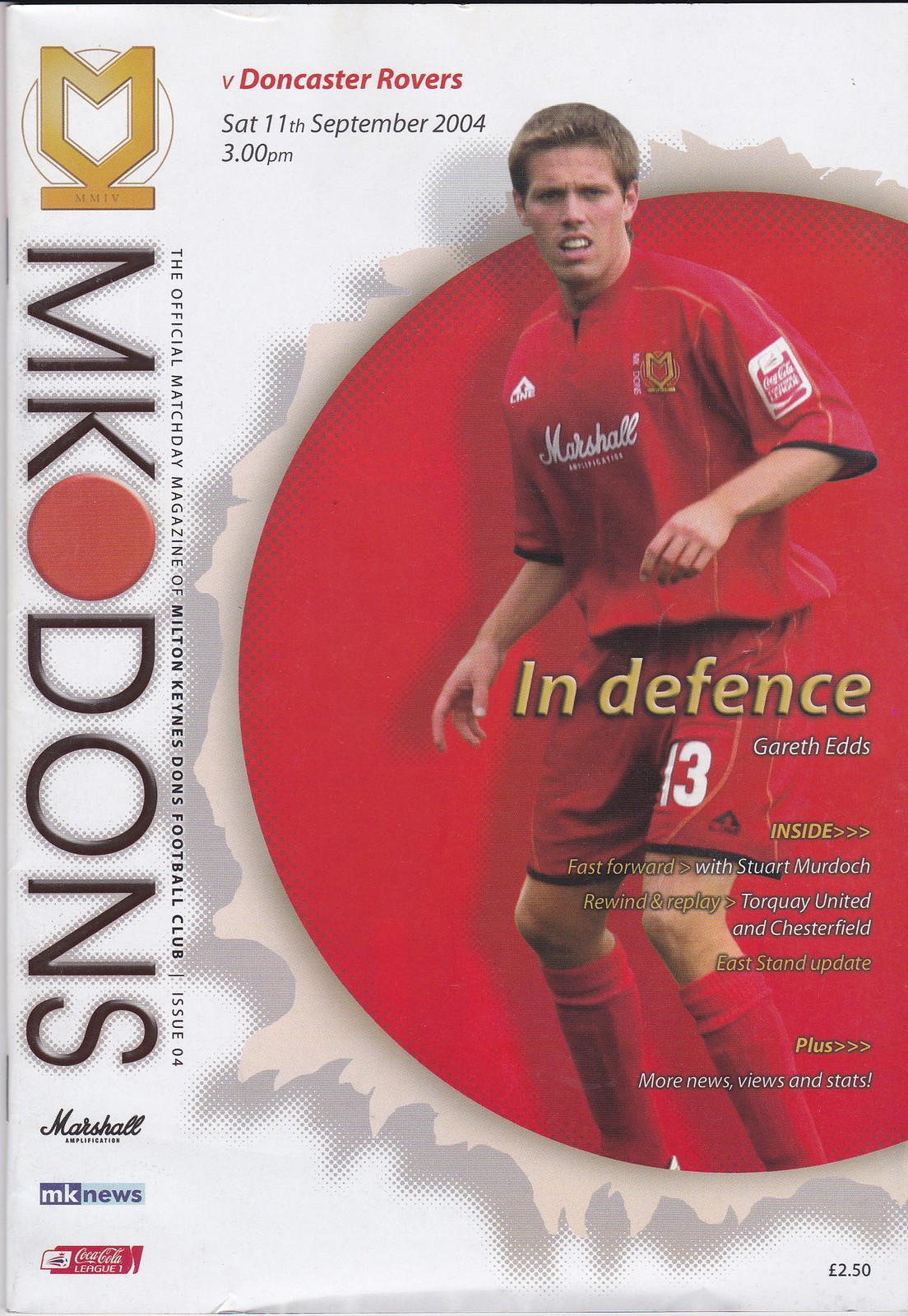This is the cover of a vertical rectangular program from a soccer match held on Saturday, September 11, 2004, at 3:00 PM. The background of the program is white with some gray accents adding texture. A large red circle dominates the center, with a soccer player superimposed over it. The player, who appears to be number 13, wears a red uniform consisting of a short-sleeved jersey, shorts, and socks, all emblazoned with the sponsor name "Marshall" on the front of the jersey. Down the left side of the cover, the word "MecoDons" is written vertically. At the top, the program states "Doncaster Rovers," indicating the opposing team. Additional text describes the program as the official Match Day magazine of Milton Keynes Dons Football Club, issue 04. The cover also mentions "In defense, Gareth Eades," and inside features such as "Fast forward with Stuart Murdoch," "Rewind and replay: Torquay United and Chesterfield," along with "More news, views, and stats." The program is priced at £2.50. Sponsors such as MK News, Coca-Cola, and Marshall are listed at the bottom.